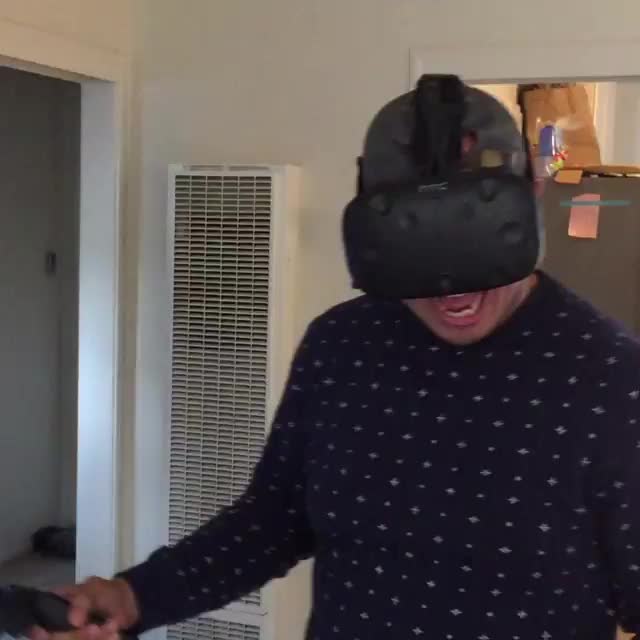This close-up photograph captures a man, appearing to be white, wearing a virtual reality (VR) headset and a hat beneath it. He is facing the viewer and is dressed in a navy blue long-sleeve shirt adorned with white speckles. His mouth is open, possibly indicating excitement or fear, with his tongue nearly hanging out. His nose and eyes are obscured by the black VR headset. His right arm, extended at waist height, clutches a VR gaming controller. The background features a white wall with a vent extending partway up, a doorway to a hallway on the left, and another room behind him. In this adjacent room, there is a tall piece of furniture with a brown paper sack on top.